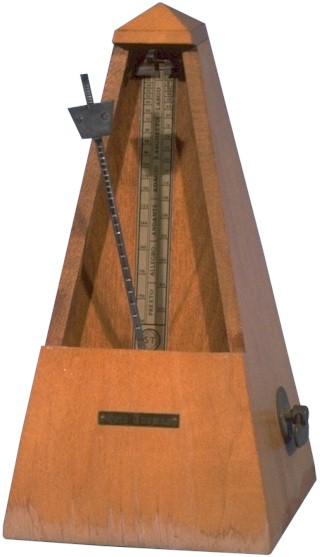The image features an intricate time-keeping device encased in a wooden box shaped like a pyramid with four distinct sides, each made from light brown wood. The entire structure tapers elegantly to a pointed apex. Captured from a front-facing perspective, the centerpiece of the device is an upside-down pendulum suspended from its midpoint, extending upward with a large trapezoidal weight attached slightly off-center, indicative of its ticking motion. A prominent white strip runs vertically down the center of the timepiece, adding contrast to the design. A shadow of the pendulum is cast on the back panel of the pyramid, enhancing the perception of depth. At the base of the device, there is a black label or plaque, though the inscription is illegible. To the right side of the wooden base, there is a dark metal circular latch or handle, suggesting portability.